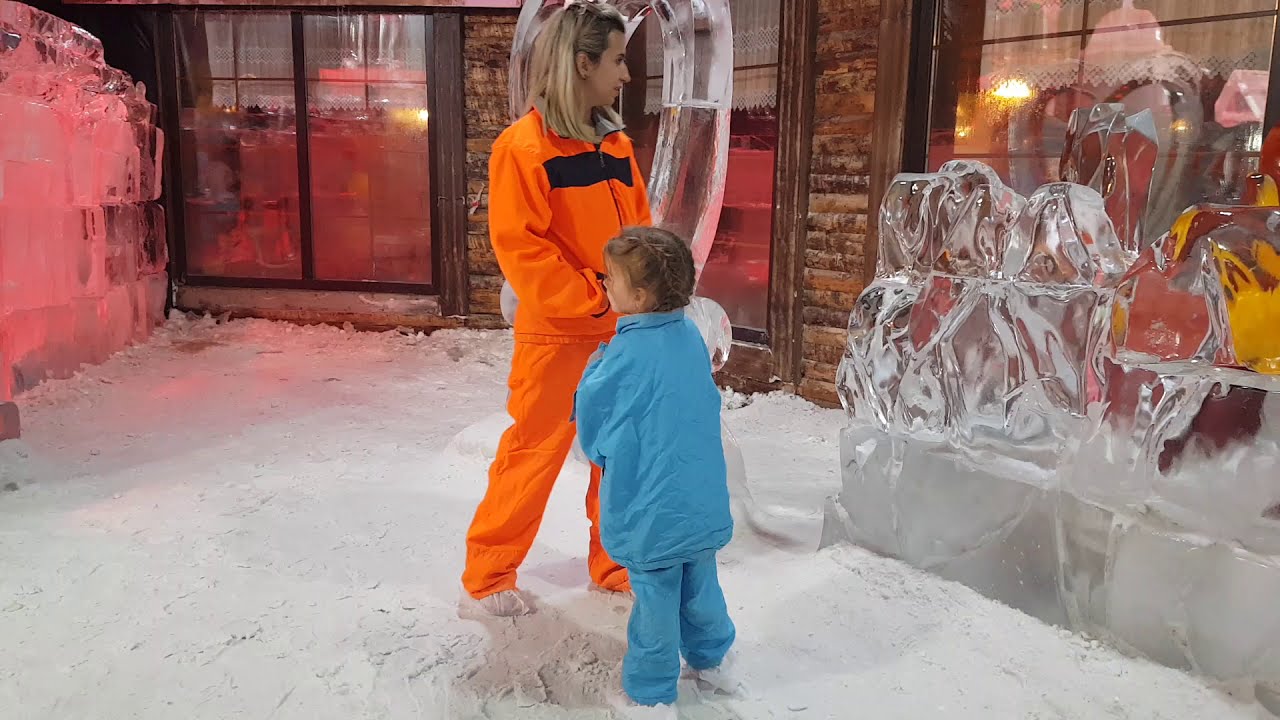In the photograph, a woman and a young girl are standing amidst what appears to be snow or a white powdery substance, possibly in front of a wooden structure resembling a log cabin. The woman, who has blonde hair that falls just past her shoulders, is dressed in a vibrant orange jumpsuit with a distinctive black stripe across the chest. Her head is turned to the right, gazing downward at a close-by ice sculpture. She also appears to have glasses or a headband atop her head and is wearing white linen covers over her shoes.

In front of her and reaching up to her stomach level stands a young girl with braided brown hair. The girl, sporting a blue jacket and pants, is facing left, towards another ice sculpture. She, too, has white linen shoe covers. The background is adorned with multiple ice sculptures: a circular one partially blocked by the woman, a more elaborate crystalline sculpture with three lumps on top to the far right, and a round one in the far left corner. The ice sculptures are strategically positioned near the building, which features a large window with a black frame, divided by lines, one window letting through a pinkish light from the left and another emitting brighter orange light from the right.

The scene conveys a striking contrast between the warmth of the indoor lights and the cold, icy exteriors, capturing a tender moment between the woman and presumably her daughter as they admire the intriguing ice sculptures.